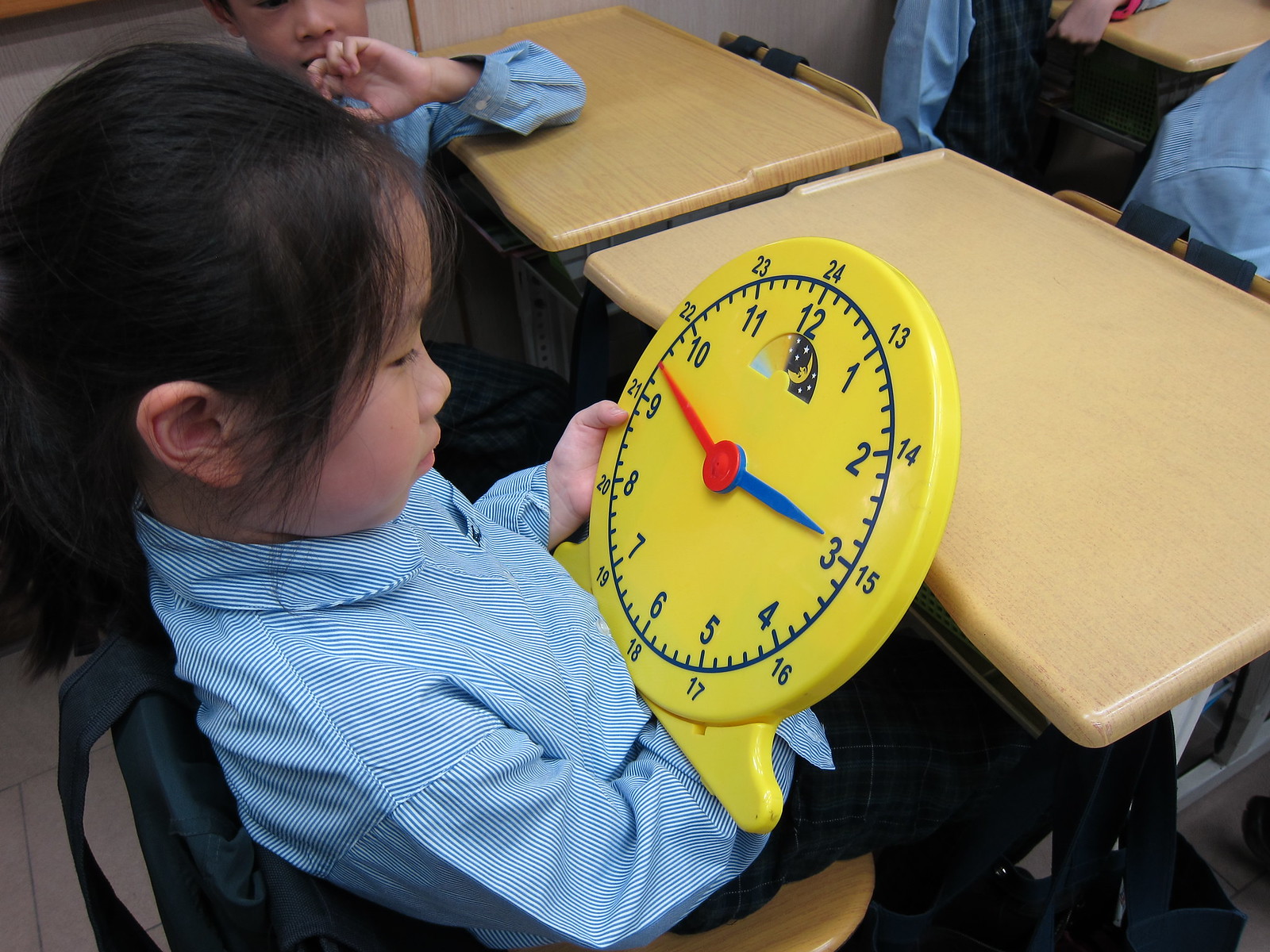In a bustling school setting, a young Asian girl with black hair tied back sits attentively at a light brown wooden desk. She is dressed in a blue and white vertically striped button-up long-sleeved shirt, matching her classmates around her. Her shirt features collars and cuff buttons, giving a neat and uniform appearance. Seated beside her are other children in similar attire, with the back of their shirts visible as they occupy desks in a staggered arrangement.

The focal point of the image is the bright yellow plastic clock that the girl is holding with her left hand, her right hand supporting it from behind. The clock, likely a learning tool for telling time, is detailed with blue numerals around its dial. The hour hand is short and blue, while the minute hand is longer and red. The clock face displays the time as 2:57. Additionally, there is a small cut-out at the top of the clock beneath the number 12, showing a glimpse of a moon image, indicating perhaps the day and night cycles.

The girl's focus is on this educational clock, suggesting a moment of learning. The clear structure and vibrant colors of the tool, alongside the attentive posture of the child, capture a snapshot of engaged learning in a classroom environment.